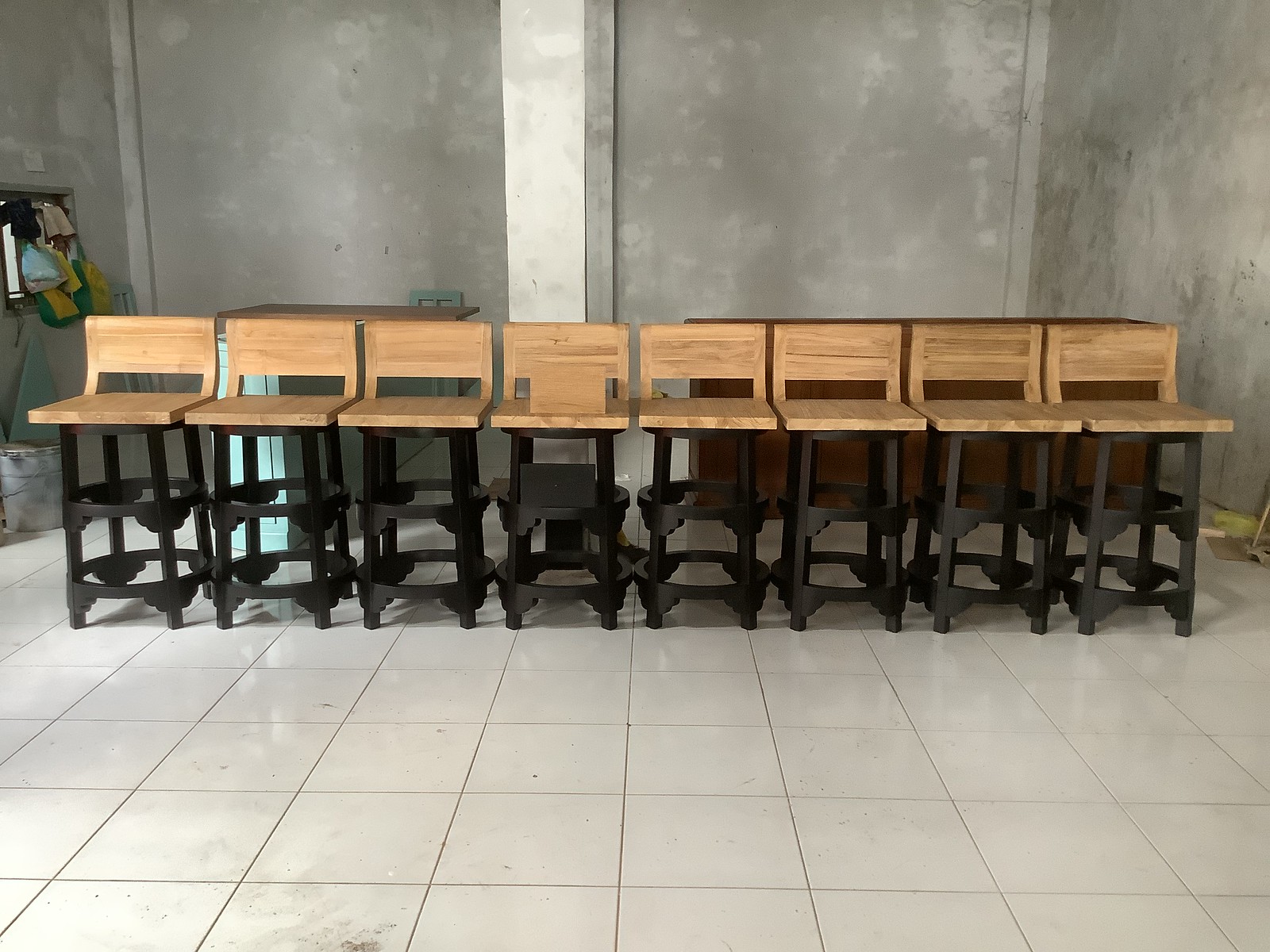This photograph captures a row of uniquely designed bar stools made of timber wood, each aligned side by side with minimal backrests. The stools feature a circular base with three circular rails connecting four black legs, and the seats comprise a flat wooden slab with a slight curved slab for support. Despite their high stature, the stools have short backs that provide limited support, echoing the construction detail described and highlighted by all observations.

One standout stool located centrally bears a distinctive brown letter, contrasting with the otherwise uniform appearance of the stools. The setting includes a grey wall adorned with a white pillar and white tiled flooring. A metal bucket, along with green and yellow objects, is visible on a grey windowsill to the left side of the scene. Additionally, the background showcases various cabinets: a brown one to the right, and a combination of blue, green, and brown furniture pieces to the left. The carefully arranged scene implies an intentional, organized space possibly not yet open to the public.